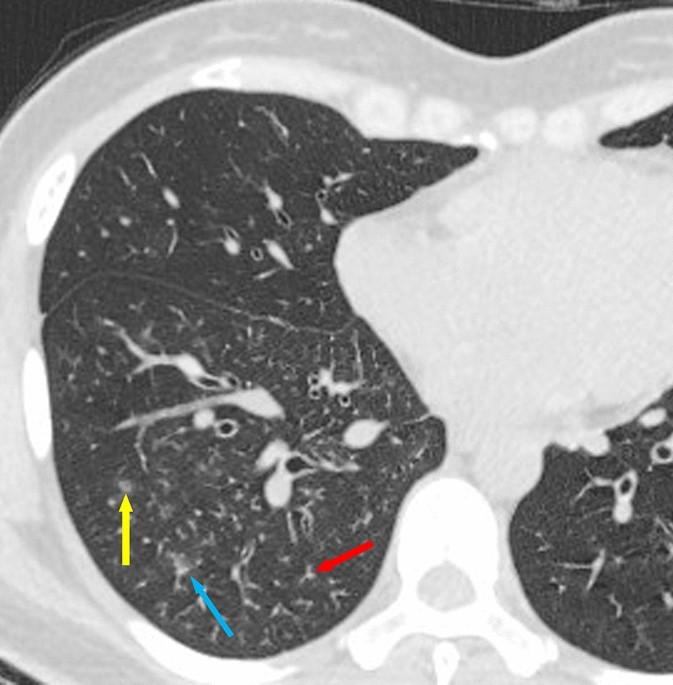This black and white medical scan, possibly a CT scan or X-ray, contains several detailed elements for educational or diagnostic purposes. The central area, filled with numerous white spots against a dark background, suggests an internal part of the human body—potentially the brain or lungs. Identifiable structural elements resemble the spine's shape at the bottom of the image. Scattered across the scan are three colored arrows—red, blue, and yellow—each pointing to specific small white spots, indicating areas of interest or abnormality. Despite the absence of explanatory text accompanying the arrows, the scan serves a critical role in medical education or patient diagnosis.